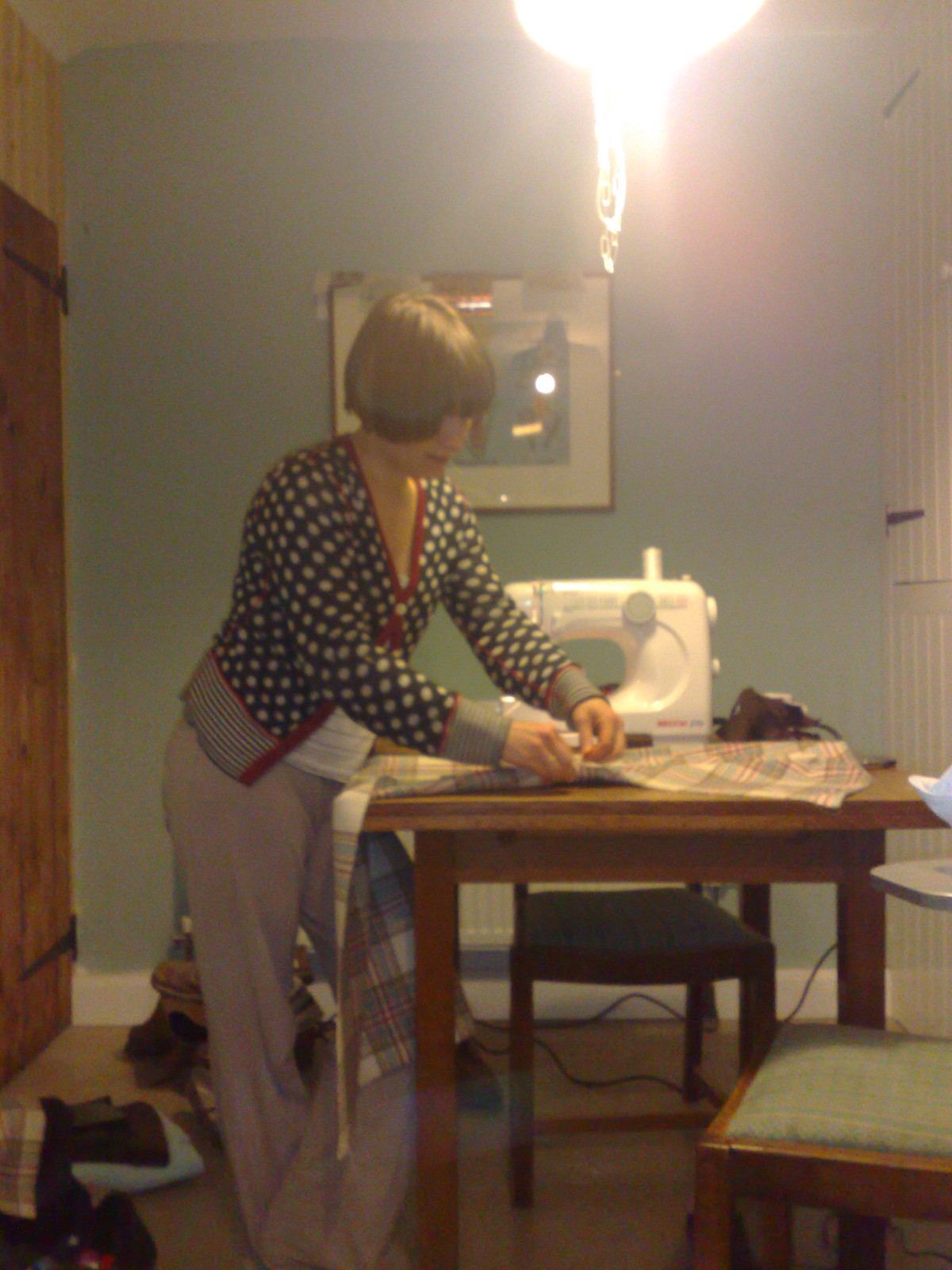This detailed color photograph captures a focused woman in a home sewing room. She is standing in front of a brown wooden table, bent slightly over her white sewing machine, diligently working on a piece of fabric. With short, bobbed hair that appears to be a mix of brown and blond, she is dressed in a distinctive black sweater adorned with white circles and a red lining, paired with beige slacks. The table holds the large sewing machine with a green handle on its left side and has two chairs, one scarcely visible behind the table and the other, a wooden chair with green upholstery, in the lower left corner of the image. Behind her, stacks of additional materials rest on the floor, suggesting future projects. The room's light green wall features a dresser and a picture frame, adding to the cozy, homely atmosphere of the sewing space.